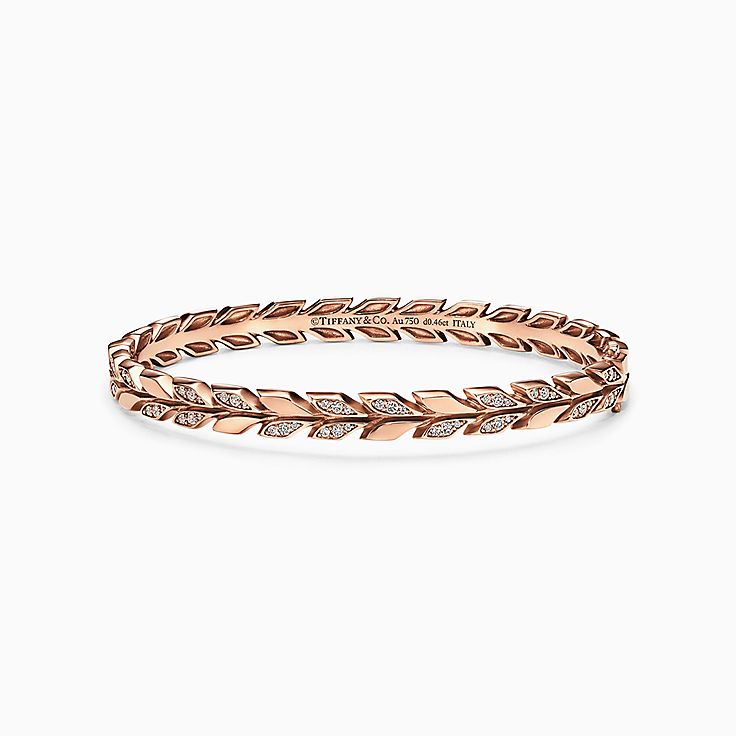The photograph showcases a bracelet set against a pristine white background. The bracelet appears to be crafted from rose gold, though it could potentially be platinum or another metal. The design features an intricate pattern of stylized, leaf-like or arrow shapes, with some segments encrusted with tiny diamonds or gemstones. Engraved on the inner side of the band are the inscriptions: "Tiffany & Co," "AU 750," ".46 carat," and "Italy," indicating its maker, material, and origin. The meticulous arrangement of the decorative elements adds both elegance and complexity to the piece, highlighting its luxurious craftsmanship.